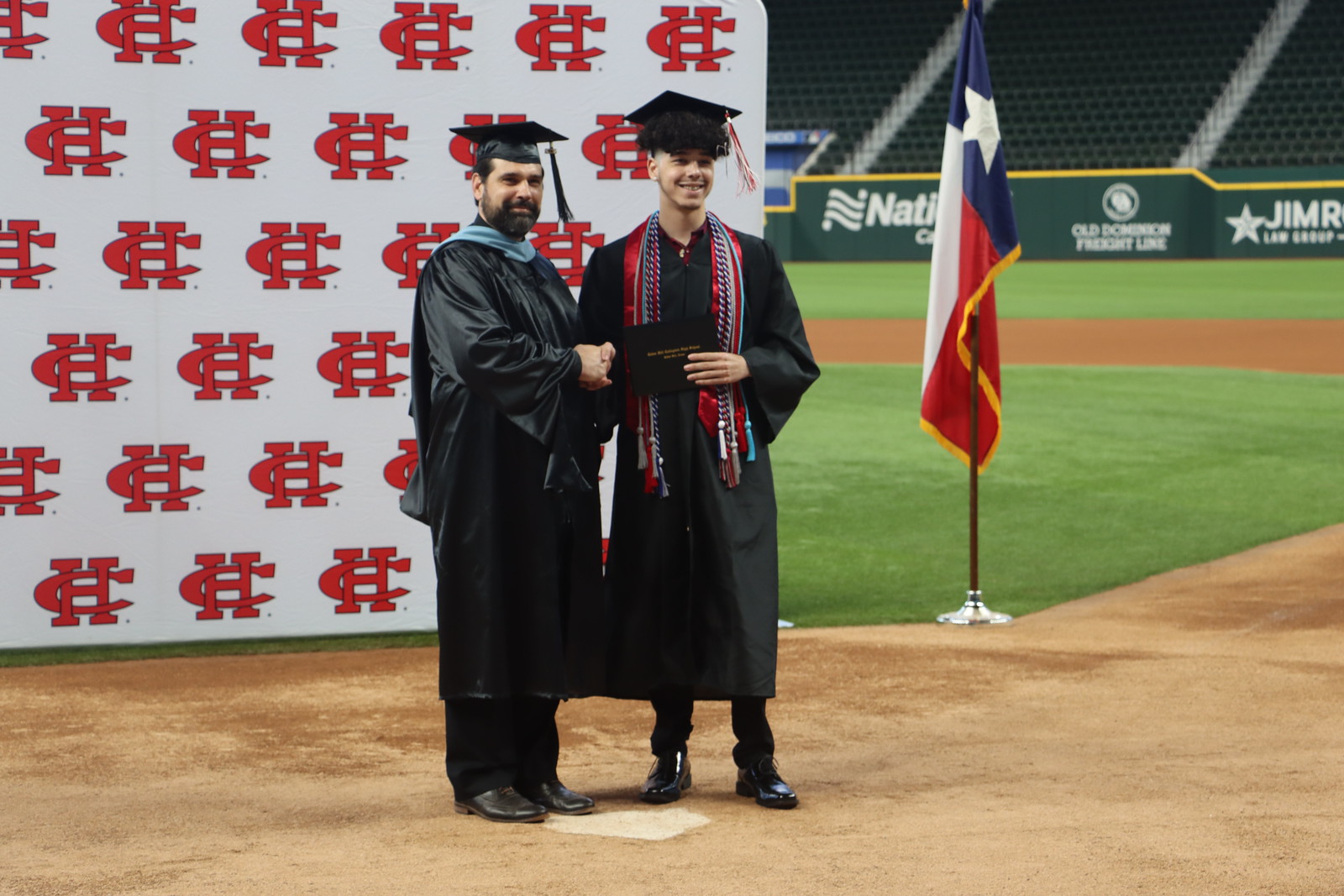This image depicts a graduation ceremony set on a baseball field, with two men standing near home plate in full academic regalia, including black gowns, mortarboards, and black shoes. The man on the left is likely presenting an award or diploma to the man on the right, who is adorned with various sashes and ceremonial honors indicative of his graduate status. Both men appear to be shaking hands as the graduate holds his diploma.

Positioned in the top left of the image, there is a backdrop featuring a series of red logos on a white background, arranged in diagonal rows showing an "H" intersected with a "C". Adjacent to this backdrop stands a flagpole with a black, white, and red state flag bearing a white star on the black portion. Behind the flagpole are the green bleachers designated for spectators, with a green barrier in front that displays promotional material from sponsors such as National Car Rental and JMR. The baseball field’s grass is neatly maintained, and the overall setting highlights a moment of academic celebration infused with a sporting venue's ambiance.